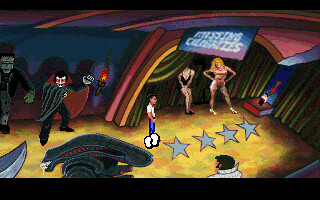This image appears to be a still frame from a cartoon or a video game, featuring a vibrant array of colors including reds, blues, pinks, grays, oranges, yellows, blacks, and whites. It is framed with a black border at the top and bottom, suggesting it's a screen capture from a video. 

On the left, a vampire character is depicted with a white face, black cape with red lining, and dark attire, alongside a green-faced Frankenstein figure. To the right of the monsters, a child with a white t-shirt, blue pants, and large white shoes stands. Beneath them on an orange and multicolored floor, four gray stars are laid out.

The scene transitions to the right where two female characters are positioned under a banner reading “Missing Celebrities,” suspended from an archway with curtains resembling a pavilion. One woman wears a black t-shirt, while the other is dressed in a pink leotard with white shorts. In the bottom right corner, the backside of a person with black hair and a gray shirt is visible, possibly reminiscent of Elvis Presley. The detailed amalgamation of cartoonish elements creates a rich, dynamic scene.